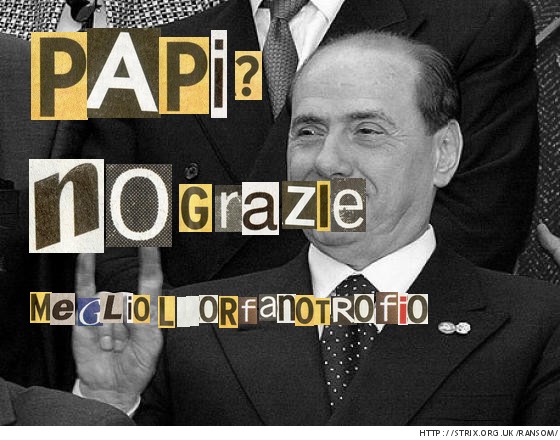This wide rectangular black and white image features Silvio Berlusconi, the former Prime Minister of Italy, prominently positioned on the right side, visible from the shoulders up. He is an older, balding man with dark hair, clad in a black suit, white button-up shirt, and a striking black tie adorned with white polka dots. In the bottom left corner, his hand is visible, forming a horned sign with his two middle fingers bent down. The collage-like text in the top left corner reads, "PAPI?" with each letter in a different color and background: the P's are green on gold, the A is white on green, and the I is black on white. Below this, in a similar ransom-note style, it reads, "NO GRAZI MAGLIO LORFANO TROPIO." In the background, other blurry figures in suits suggest a formal setting. Berlusconi's confident, somewhat smug expression adds to the meme-like quality of the image. The mixed-font and magazine-cutout style letters contribute to the mysterious and eclectic vibe.